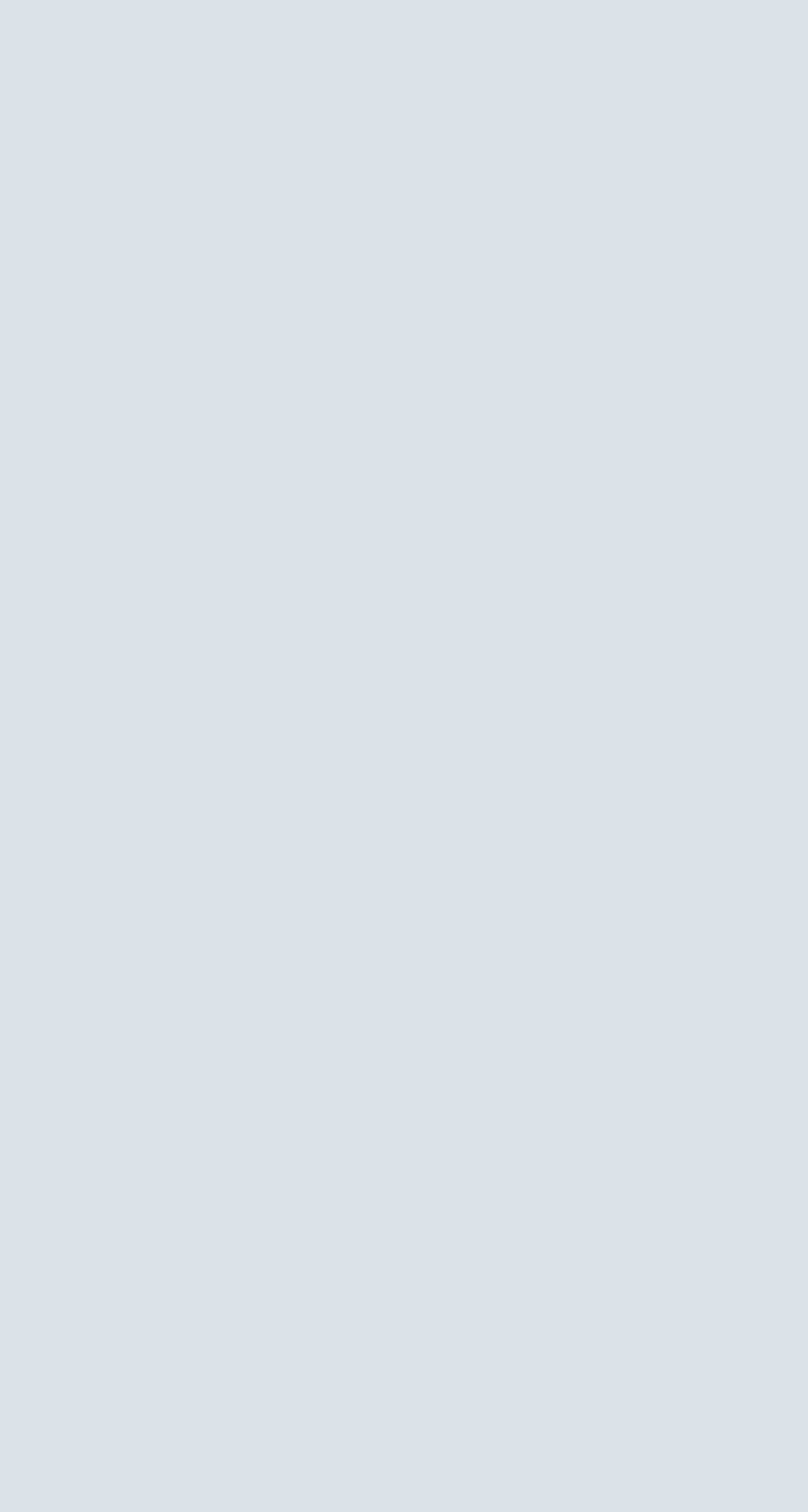A vertically oriented, medium-sized rectangular box dominates the frame of this image. The background is uniformly filled with a light gray color, giving it a stark, minimalist appearance. The edges of the rectangle are sharply defined, not rounded, emphasizing its geometric precision. The shorter sides of the rectangle, situated at the top and bottom, contrast with the longer vertical sides on the left and right. The image is devoid of any elements or apps, presenting a clean and unembellished expanse of light gray. There is no discernible border, making the entire rectangle appear as a singular, continuous light gray box, with the shorter sides measuring approximately two to three inches in length and the longer sides extending a few inches more.